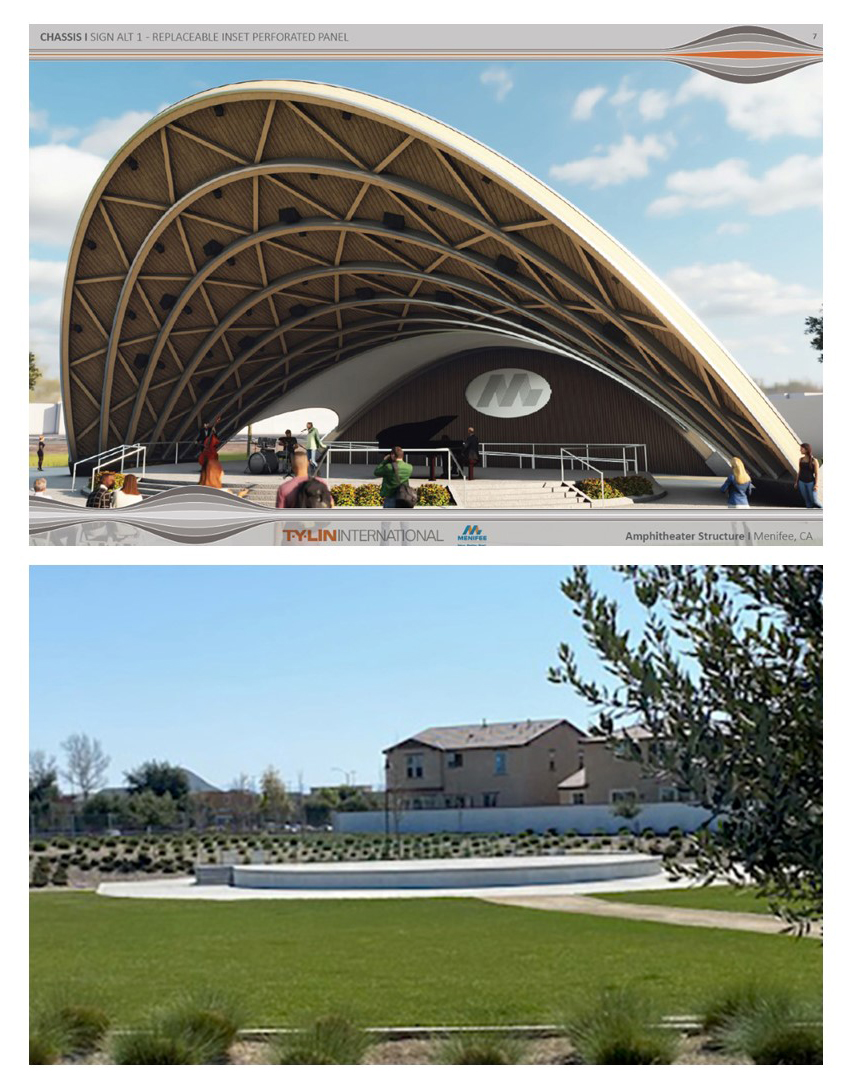The image consists of two distinct pictures. 

The top picture appears to be of an amphitheater-like structure. In the foreground, several people can be seen standing, while a few others are seated towards the left, though they are partially obscured. Prominent stairs lead up to another area, but the view is restricted by distance. At the far end, an "M" on an oval sign hangs beneath a large arch, reinforcing the amphitheater impression. The arch itself is intricately designed with six rows of zigzag patterns adding to the architectural detail.

The bottom picture depicts a garden scene. The garden features various elements including seating areas, a variety of bushes and different types of plants organized into beds. In the background stands a two-story house, painted beige, complementing the lush green of the garden.

Together, these pictures juxtapose architectural magnificence with natural tranquility.